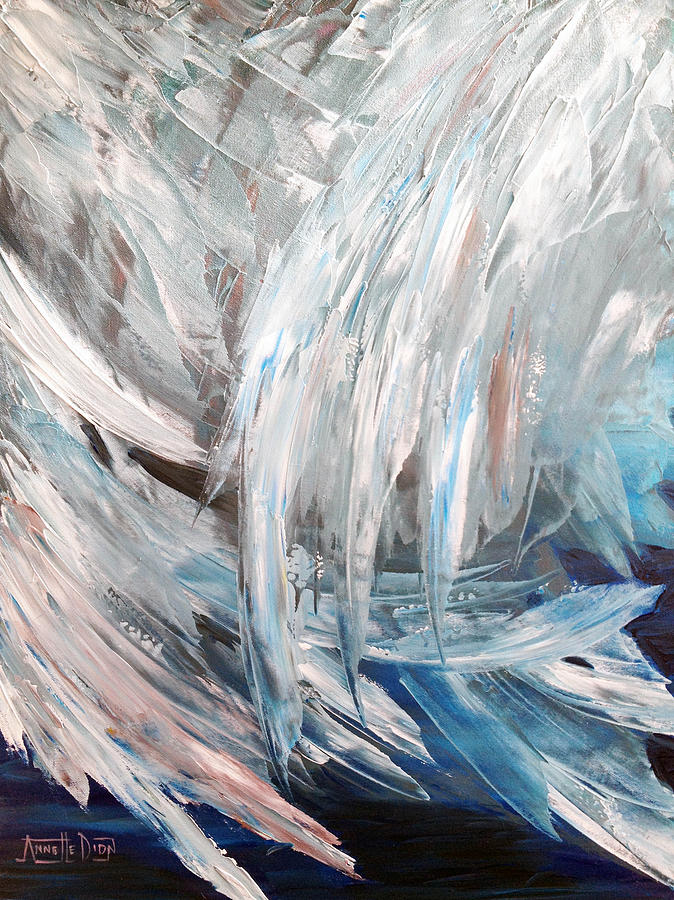The image is a vertical, abstract painting that prominently features overlapping wing-like structures rendered in sweeping, palette-knife strokes. These wings, likely representing either angel or swan wings, exhibit a primarily white color palette interspersed with light blue and gray hues for depth. The largest wing curves from the upper right towards the middle, with additional smaller wings adding a sense of layered texture. The background transitions into darker shades, with the lower section featuring black and dark blue tones, lending an almost underwater ambiance to the piece. In the bottom left corner of the painting, there is a peach-colored signature that is partially legible, possibly reading "Annette Dione" or "ANHEIDIN," although it's difficult to be certain. The overall composition elegantly captures the ethereal and dynamic essence of the wings.